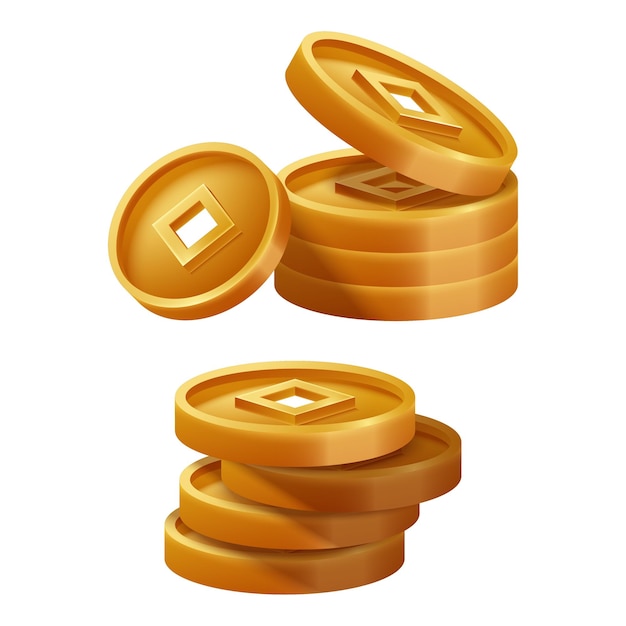The image features a collection of round, dark gold-colored discs, distinctively designed with a square cutout in the center through which white space is visible. The composition contains two separate stacks of these discs set against a plain white background. At the bottom, there are four discs stacked together, each slightly misaligned to reveal the square cutouts prominently. Above these, there is another group featuring five discs: three are neatly stacked, one at the top is tilted from right to left, and a separate disc leans against the stack. The symmetrical arrangement and unique design of the discs, coupled with the stark background, draw attention to their intriguing square-centered cutouts.